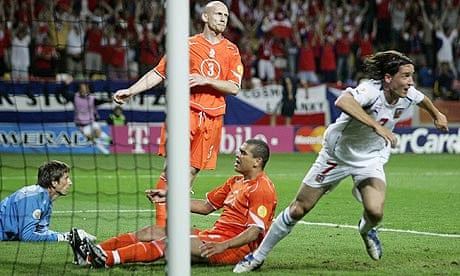In this vibrant photograph of a professional soccer game, the action is set against the backdrop of a full stadium brimming with cheering fans, their raised hands capturing the excitement of an ongoing match. The scene on the green pitch features four main players: two in bright orange uniforms with matching jerseys, shorts, and socks, one in a white uniform accented with red details, and a goalie in a long-sleeve, light blue shirt with brown hair, who is seated on the ground to the left. The goalie appears to be of Hispanic descent, notable by his dark skin tone.

The player in white seems to be running away from the net to the right side of the picture, suggesting that a goal may have just been scored. The image prominently includes the left side of the net, identifiable by its white posts and see-through black mesh, positioned near the center vertical of the frame. Surrounding the pitch is a collection of colorful sponsor banners, including a visible T-Mobile ad in purple, adding to the professional atmosphere of the scene.

Overall, the dynamic composition and the enthusiastic support of the crowd, along with the detailed players' uniforms and strategic advertisement placements, effectively convey the high stakes and intense emotions of a professional soccer match in progress.